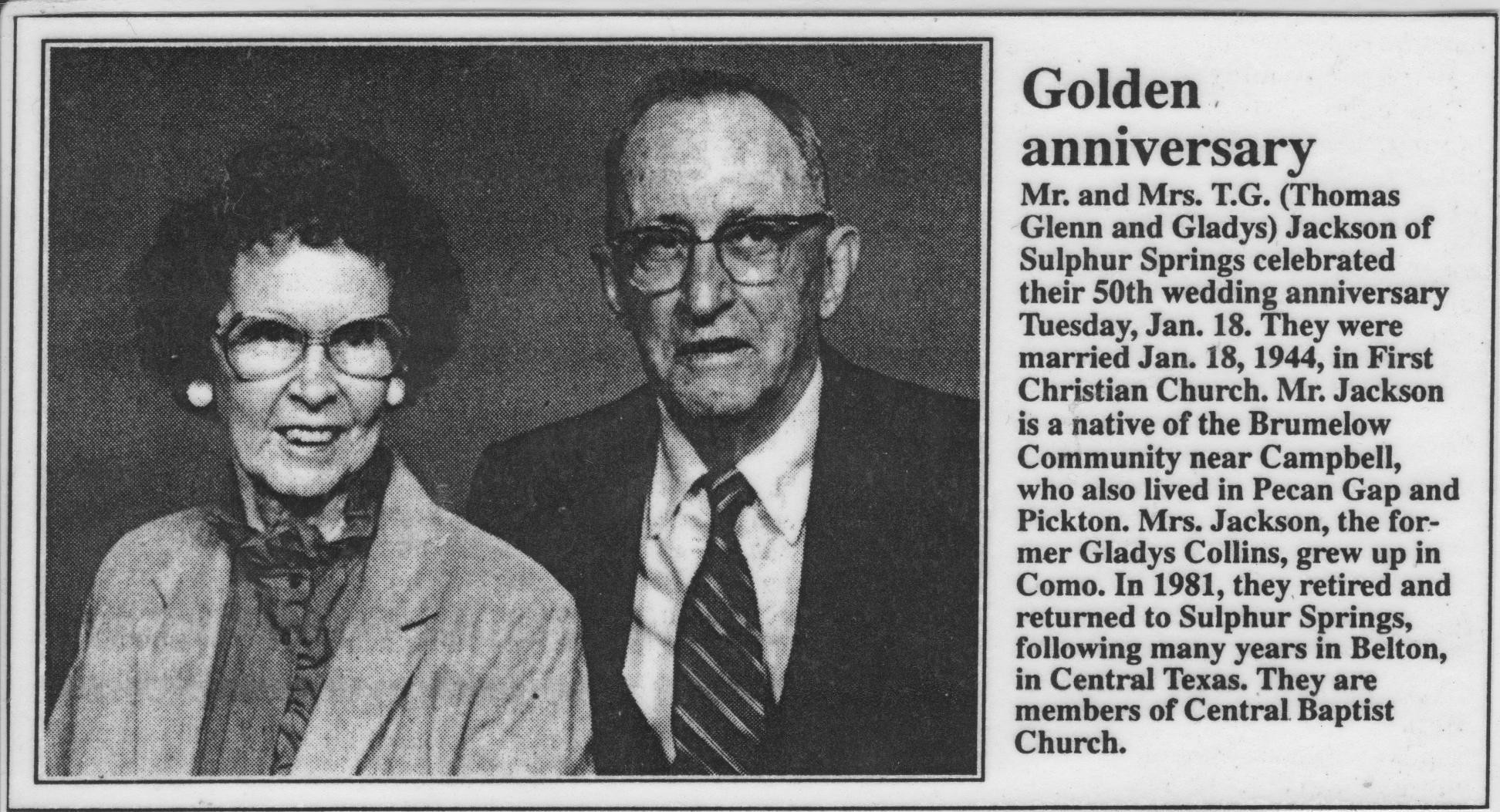This black-and-white newspaper announcement, featuring a detailed celebration of Mr. and Mrs. T. G. (Thomas Glenn) and Gladys Jackson's 50th wedding anniversary, is divided into two sections. The left two-thirds of the image displays a photograph of the couple. Mr. Jackson, dressed in a suit with a tie, stands beside Mrs. Jackson, who wears a frilly shirt with a light coat and white earrings. Both are wearing glasses. The right side of the image contains text on a light gray background, prominently featuring the bold title "Golden Anniversary." 

The announcement details that Mr. and Mrs. T.G. Jackson of Sulphur Springs celebrated their golden anniversary on Tuesday, January 18th. They were married on January 18th, 1944, at the First Christian Church. The text includes biographical notes, mentioning Mr. Jackson's origins in the Bromeloe community near Campbell, and his residence history in Pecan Gap and Picton. Mrs. Jackson, née Gladys Collins, grew up in Como. After many years in Belton in Central Texas, the couple retired and returned to Sulphur Springs in 1981. Both are members of Central Baptist Church. The announcement not only captures the couple's long-lasting union but also their lifelong journey together.